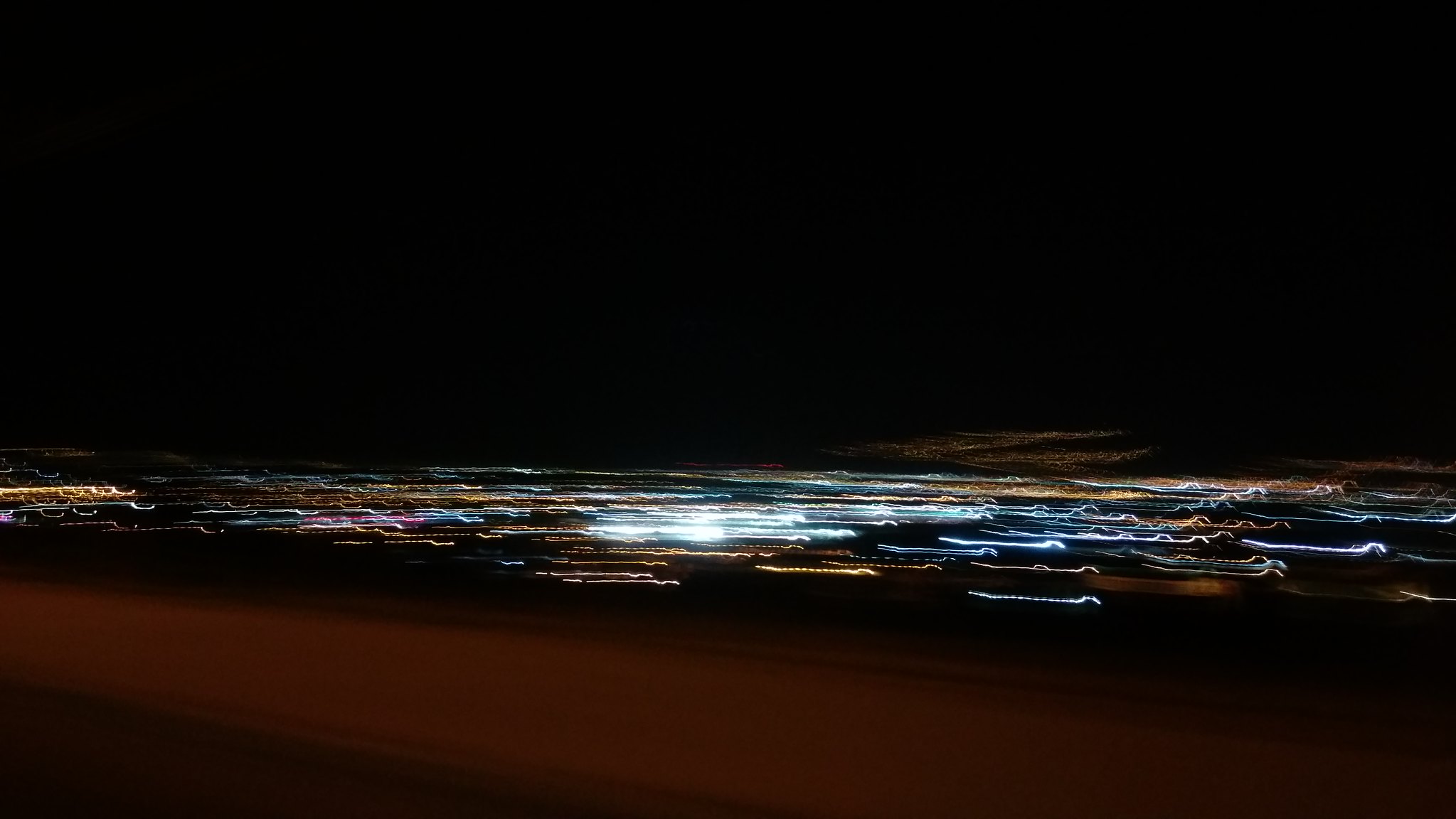A dynamic night-time cityscape captured from an elevated vantage point, showcasing the sprawling urban landscape illuminated by countless lights. The photograph features significant motion blur, transforming city lights into vibrant streaks of yellow, white, and red, crisscrossing the image. The neon trails paint an energetic tableau against a backdrop of the dark night sky, creating a striking contrast and emphasizing the bustling spirit of the metropolis.